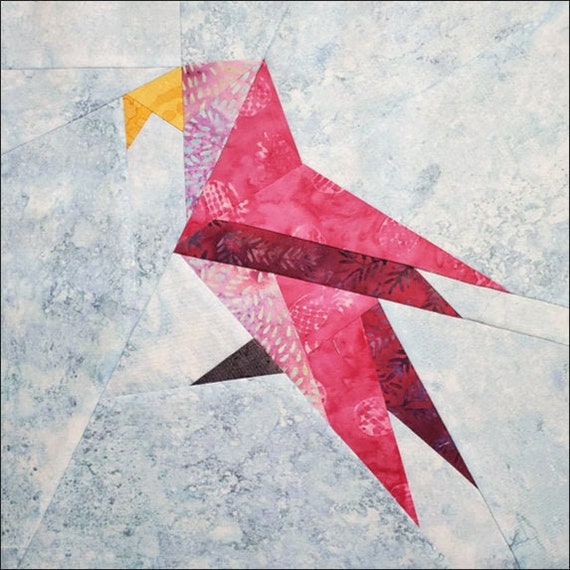The image depicts an artistic representation of a bird composed of geometric shapes, resembling an origami design. The background is a light blue-gray color, reminiscent of weathered paper or concrete, creating a stark contrast that emphasizes the central subject. The bird, prominently showcased in the middle of the image, is crafted from various shades of pink, transitioning to dark red hues, and adorned with intricate patterns. Some sections of the bird's body feature floral patterns with black vines and leaves, while others display white droplets and dashes arranged in circular formations. The bird's beak is a striking yellow, and its feet are black, contributing to the overall elaborate and textured appearance of the piece. This detailed composition merges the abstract simplicity of geometric shapes with the sophistication of detailed pattern work, capturing the viewer's attention with its vivid and meticulous design.